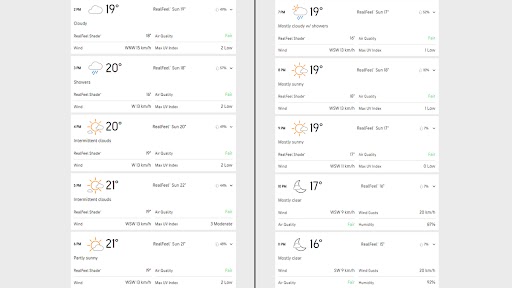This image is approximately 1.5 times wider than it is tall, with two equal halves separated by a black bar running vertically down the center. Additionally, the images are framed with gray letterboxes, accounting for about 10% of the central area and roughly 30% of the outer edges.

On the left side, the image appears to be a weather forecast. While the text is too small to read clearly, there are various weather icons and temperatures displayed. It shows five different weather conditions: 
- A cloud with 19 degrees.
- A cloud with rain and 20 degrees.
- A sun partially obscured by clouds with 20 degrees.
- A sun with 21 degrees.
- A sun with a cloud and 21 degrees.

The right side similarly displays weather conditions, which seem to be:
- A rain cloud with a sun behind it and 19 degrees.
- A sun with 19 degrees.
- Another sun with 19 degrees.
- A moon with 17 degrees.
- A moon with 16 degrees.

Overall, the image presents a detailed comparison of weather forecasts, segmented neatly into two sections with equal visual weight.